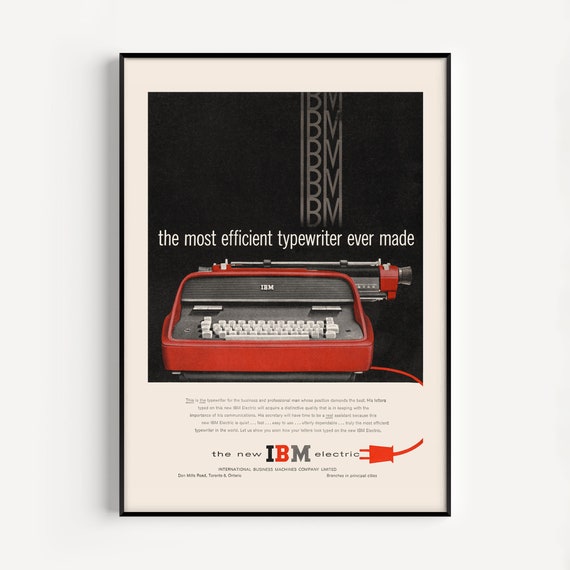This framed vintage poster, set against a white wall, prominently features a classic black electric IBM typewriter with a red plug. Housed within a sleek black frame, the poster has a main black square section emblazoned with a faded vertical "IBM" pattern repeated five times. In white text across the middle, it declares, "The most efficient typewriter ever made." Below this slogan, there's a striking image of a red IBM electric typewriter featuring white keyboard letters and a gray interior. The bottom portion of the poster displays more black text and ends with the bold inscription, "The new IBM Electric." The red plug from the typewriter is artistically connected to this text, emphasizing the innovative design. The entire scene, reminiscent of magazine ads from the 1960s, captures the elegance and technological advancement of the era.